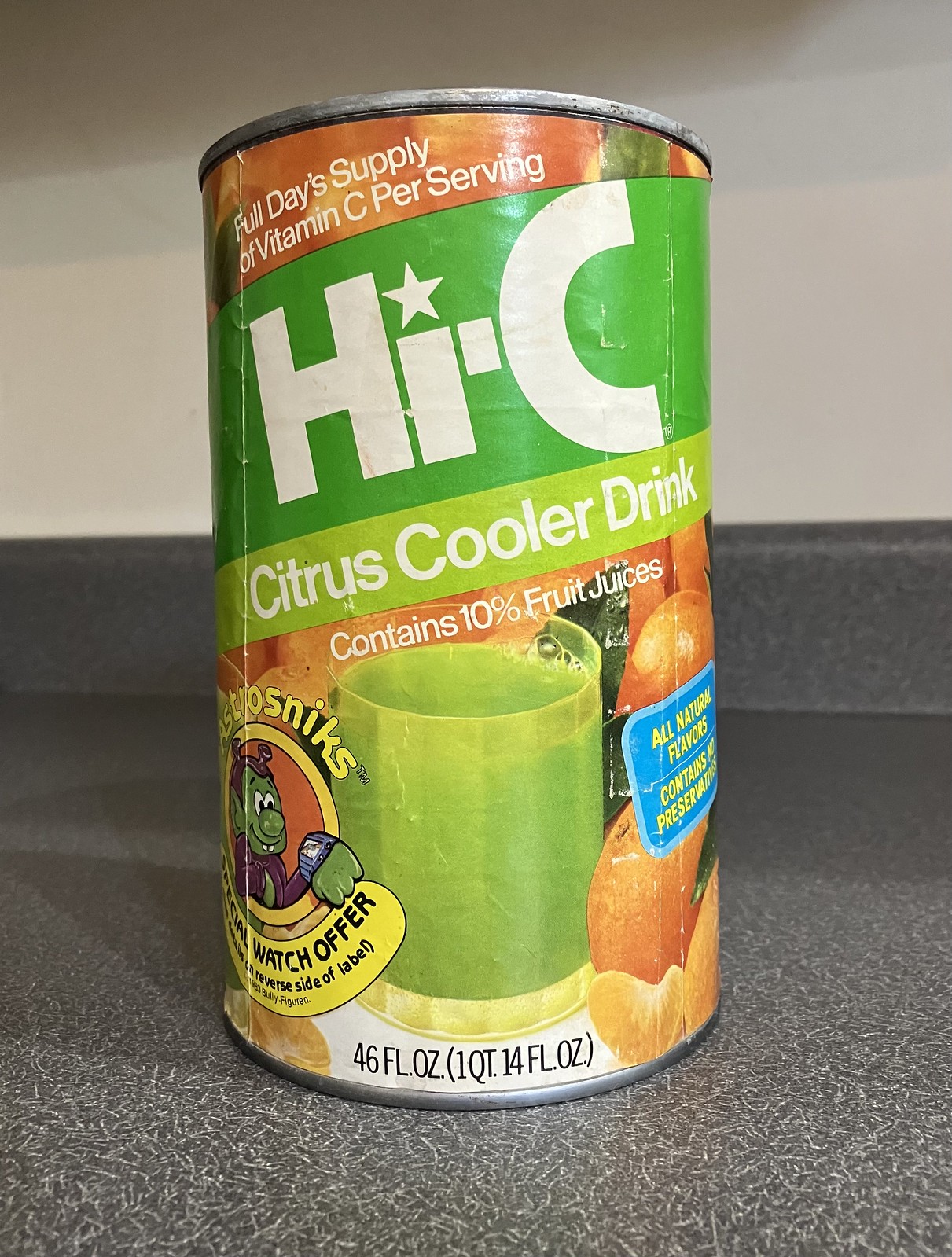This photograph features a vintage can of Hi-C fruit juice prominently displayed on a gray countertop. The countertop extends towards the back wall, which has a white-colored upper portion and a lower section that appears to match the gray of the countertop, creating a coherent backdrop. The can, presented in a perspective that accentuates its size, is cylindrical and reminiscent of a soup can in shape. It is predominantly green with bold white lettering that reads "Hi-C" near the top. Below the brand name, there is an illustration of a drink with green liquid, labeled "Citrus Cooler," accompanied by vibrant images of oranges. The bottom of the can indicates a volume of 46 FL ounces, suggesting a substantial size. The overall image is brightly lit, indicating it was taken indoors, and evokes a sense of nostalgia with its vintage aesthetic.